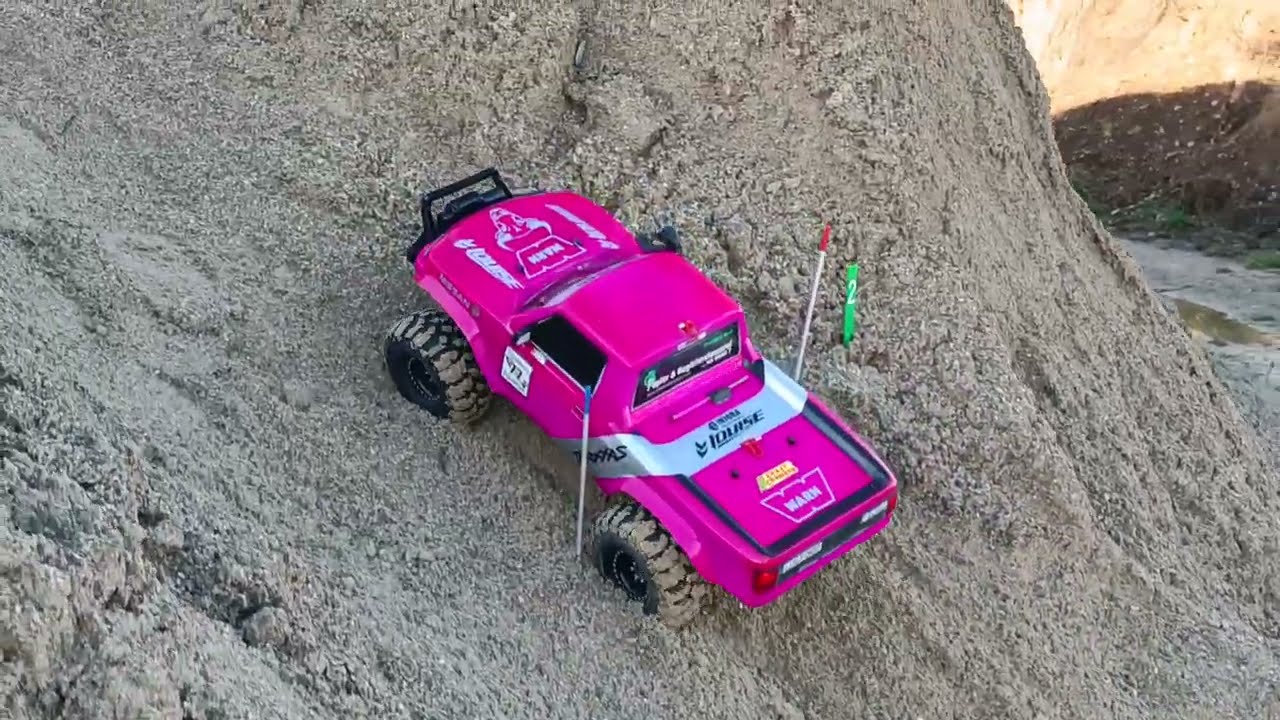This overhead shot captures a bright pink, remote-controlled (RC) truck navigating a sand pile, which appears to be a couple of feet tall and resembles a large sand dune. The close-up angle means the truck takes up almost the entire photograph, showcasing its distinct features. The truck's large black tires and plastic front push guard, equipped with a winch, suggest it's built for rugged off-road terrain. Adorned with decals, including a name that reads "Louise" and a logo that appears to say "Warm," the truck also sports a silver stripe along its back. Positioned between two small flag poles, one with a blue tip and the other with a red tip, the truck seems to be part of a slalom course, likely in a competitive setting. Tracks visible in the sand hint at prior runs. Beyond the sand pile and the immediate focus on the RC truck, a hill is discernible in the background, but no other notable landmarks are visible.